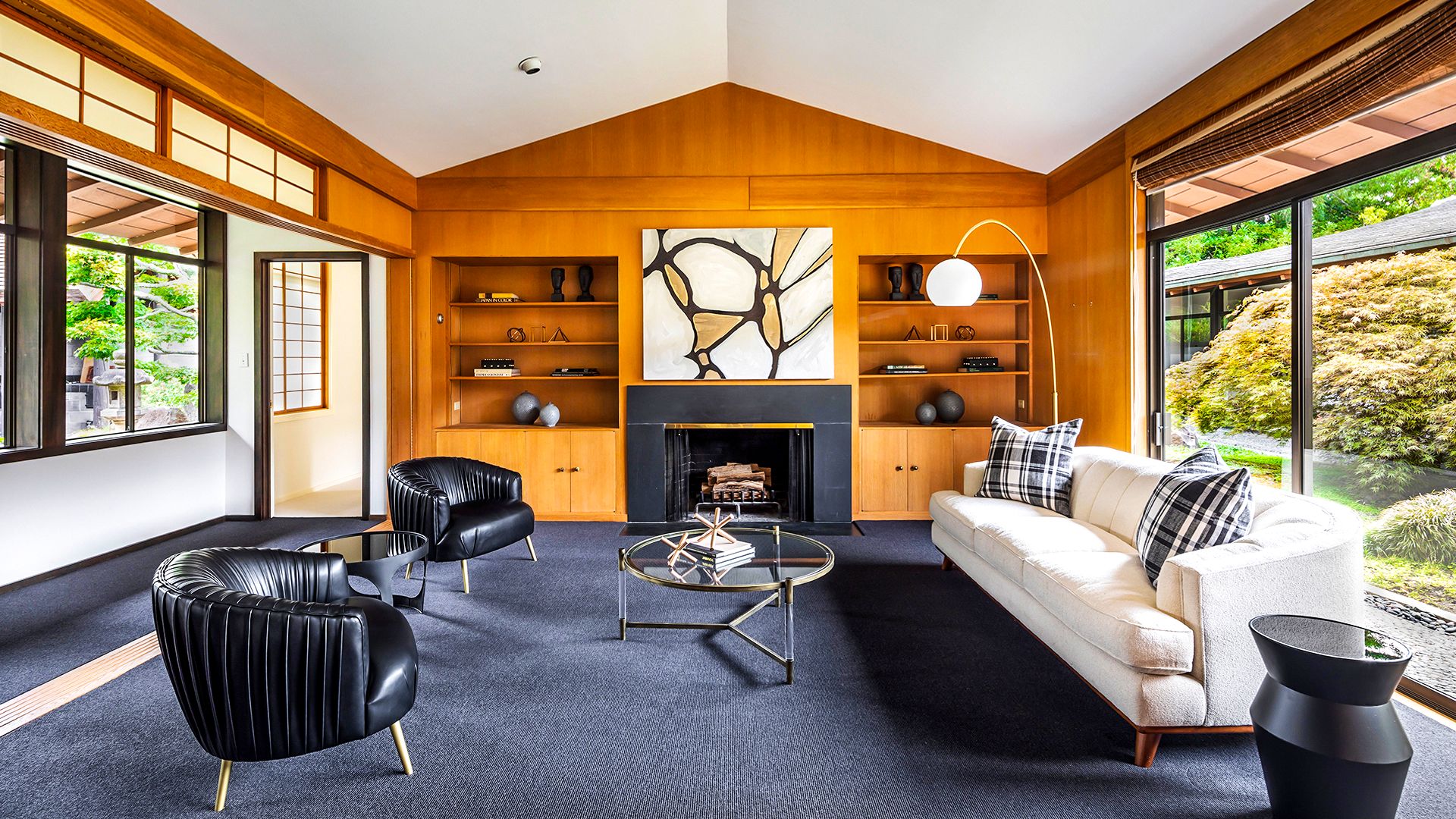This photo captures a beautifully modern and meticulously maintained living room that exudes a serene, contemporary aesthetic. The room is long and features a stunning combination of wood paneling and expansive glass windows on either side, allowing for a lush view of the well-manicured greenery outside. The ceiling is a modest cathedral style, painted white to enhance the room’s airy feel.

At the far end, a light wooden-paneled wall houses a central black fireplace adorned with a gold banner. This fireplace, which touches the floor and contains a stack of wood, is flanked by two built-in bookshelves. These shelves are filled with dark, natural-colored pottery, adding a rustic contrast to the room’s modern decor. Above the fireplace, a white and gold abstract art piece serves as a striking focal point.

The flooring is a rich blue carpet, and the seating arrangement includes two sleek black chairs with wooden legs on the left side, facing a long, ivory couch on the right. The couch is accentuated by plaid blue and white pillows on either end. A glass coffee table with decorative items and iron legs anchors the seating area, positioned between the black chairs and the ivory couch.

Overall, the interior is clean, stylish, and harmoniously blends modern design elements with warm, natural accents, creating an inviting and polished living space.